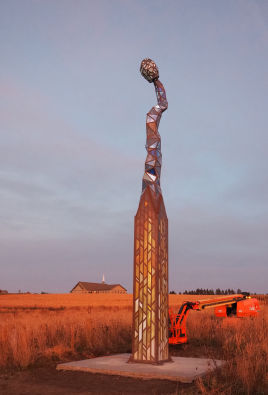The photograph captures a striking scene of an abstract, glass-like artwork standing tall amidst a vast, flat prairie landscape, possibly a wheat field. The primary focus is the intricate statue, characterized by its stained glass walls that transition from predominantly orange and brown hues at the base to shades of blue at the spire. The artwork’s design resembles an elongated structure with a crook at the top, invoking the idea of an anglerfish or an antenna-like form. This piece is centered on a gray concrete base, enclosed by a square framework.

To the right of the statue, a reddish-orange cherry picker (likely involved in the installation or maintenance of the artwork) adds an industrial touch to the serene natural environment. Extending into the background, the image includes a solemn farmhouse or church, their tan walls and brown roofs hinting at the area's rural character.

The photograph’s sky, which dominates the top half of the frame, is overcast, casting a dim, perhaps early evening or late afternoon light over the scene. This light bathes everything in a subtle orangish hue, hinting at a sunrise or sunset. The subdued colors blend with the reddish and brownish tones of the surrounding grass, creating a harmonious yet melancholic atmosphere.